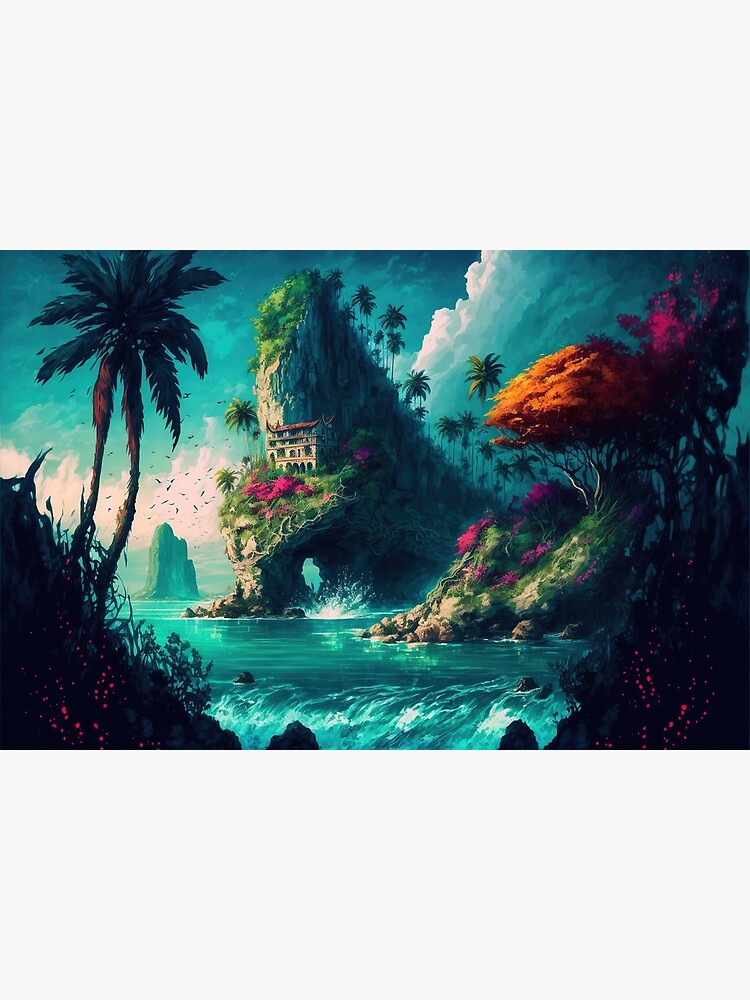A vivid, rectangular painting or computer-generated artwork, measuring approximately six inches high and four inches wide, is bordered by thick, one-inch high gray bands at the top and bottom. At the center of this frame is a dynamic scene set in a fantasy realm. A grand, multi-storied stone temple with pointed roofs stands majestically on a rocky cliff. Lush, grassy moss and clusters of pink flowers surround the temple, while tall palm trees grow behind the cliff. Below, the cliff forms cavernous openings through which water flows into a serene, light blue ocean. This ocean scene features additional rocky outcroppings rising from the water.

In the foreground, both the lower left and right corners feature dark, grassy hills dotted with pink flowers and a few palm trees. Between these hills, a waterfall cascades gracefully. The sky above is populated with large, puffy white and gray clouds and flocks of birds flying in the distance. The painting is rich with details, including multicolored trees in shades of orange and pink. This detailed and colorful depiction offers a glimpse into a fantastical, serene landscape.